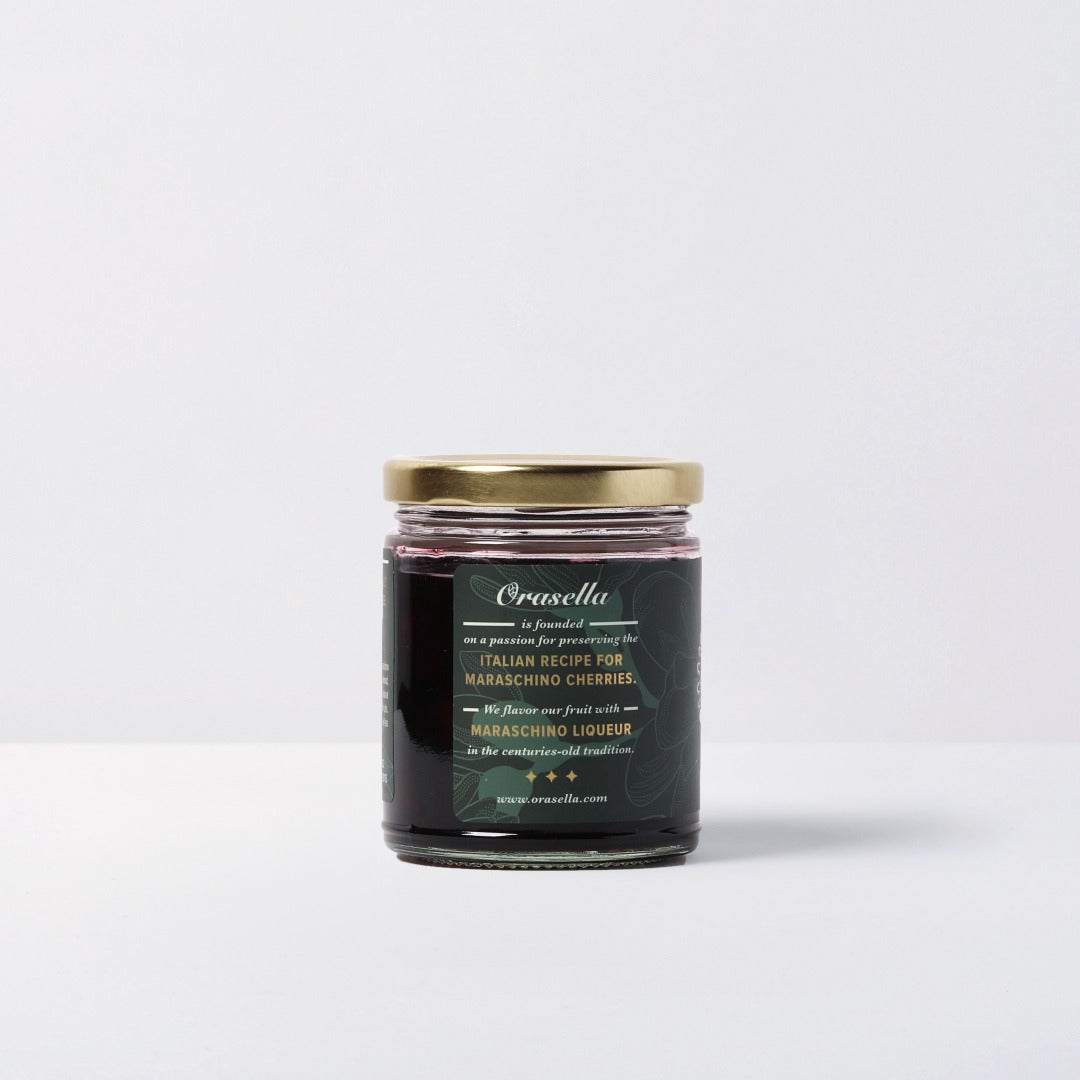The photograph showcases a small glass jar with a shiny gold lid, nestled on a white table against a white wall. The jar, labeled with a black sticker, prominently features the brand name "Oracela" in white italicized font. Beneath the brand name, a cursive inscription in white reads, "Founded on a passion for preserving." Further down, golden letters declare "Italian recipe for maraschino cherries," followed by a white statement, "We flavor our fruit with," and a gold "maraschino liqueur." The inscription concludes with "in the centuries-old tradition" and three gold diamond symbols. At the bottom, the website address "www.oracela.com" is printed in white. The jar is filled with a dark reddish liquid, which appears nearly black in the thicker portions, but reveals a hint of pinkish hue near the top. The label's background features faint green patterns, possibly leaves, adding a decorative touch. The jar's shadow is subtly reflected on the pristine white surface below.